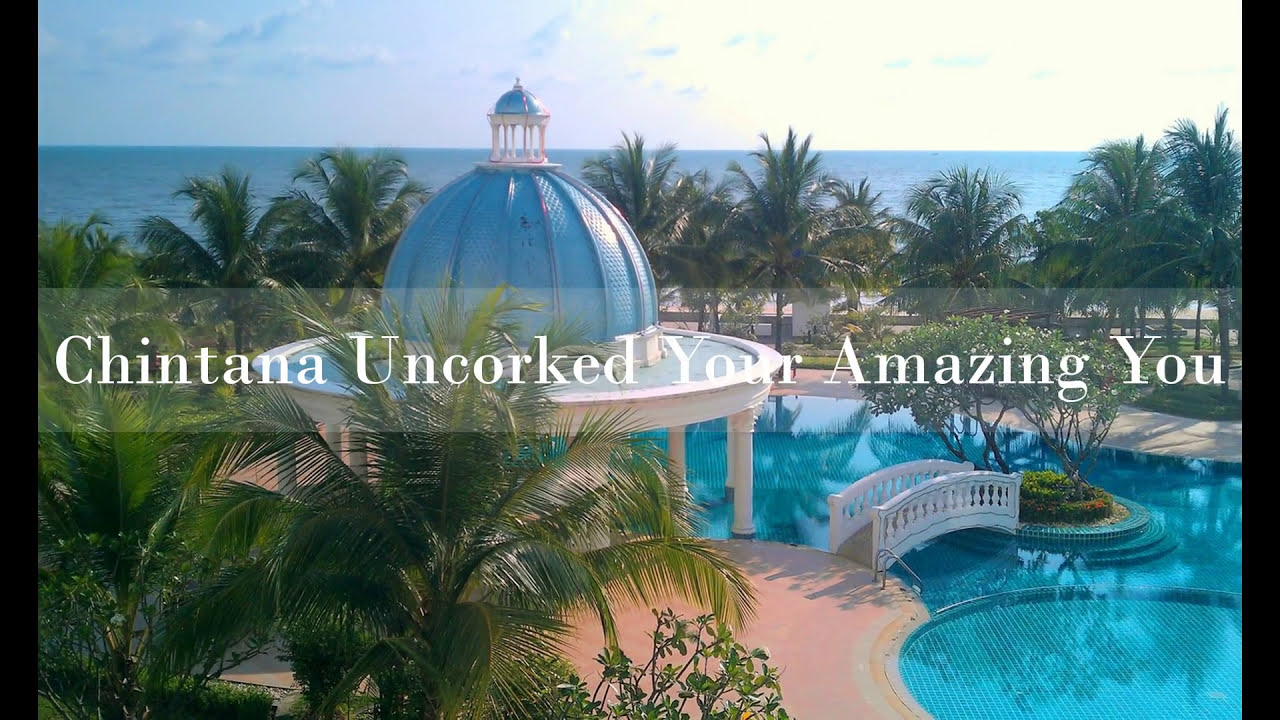The photograph captures a serene resort, showcasing a large swimming pool with bright blue water. In the center of the pool, there's a man-made island adorned with lush grass and small trees. This island is accessed via an elegant white arch bridge, which connects to a red brick sidewalk. On this sidewalk sits a prominent cabana featuring a striking blue dome and white columns, resembling a gazebo with a cupola. The entire area is framed by tall palm trees, contributing to the tropical ambiance. In the background, the blue ocean is visible just above the palm trees, meeting the sky, which is dotted with white clouds. The camera angle, approximately 15 feet off the ground, offers a comprehensive view of this picturesque setting. A transparent band across the middle of the image displays the text "Chintana uncorked your amazing you."